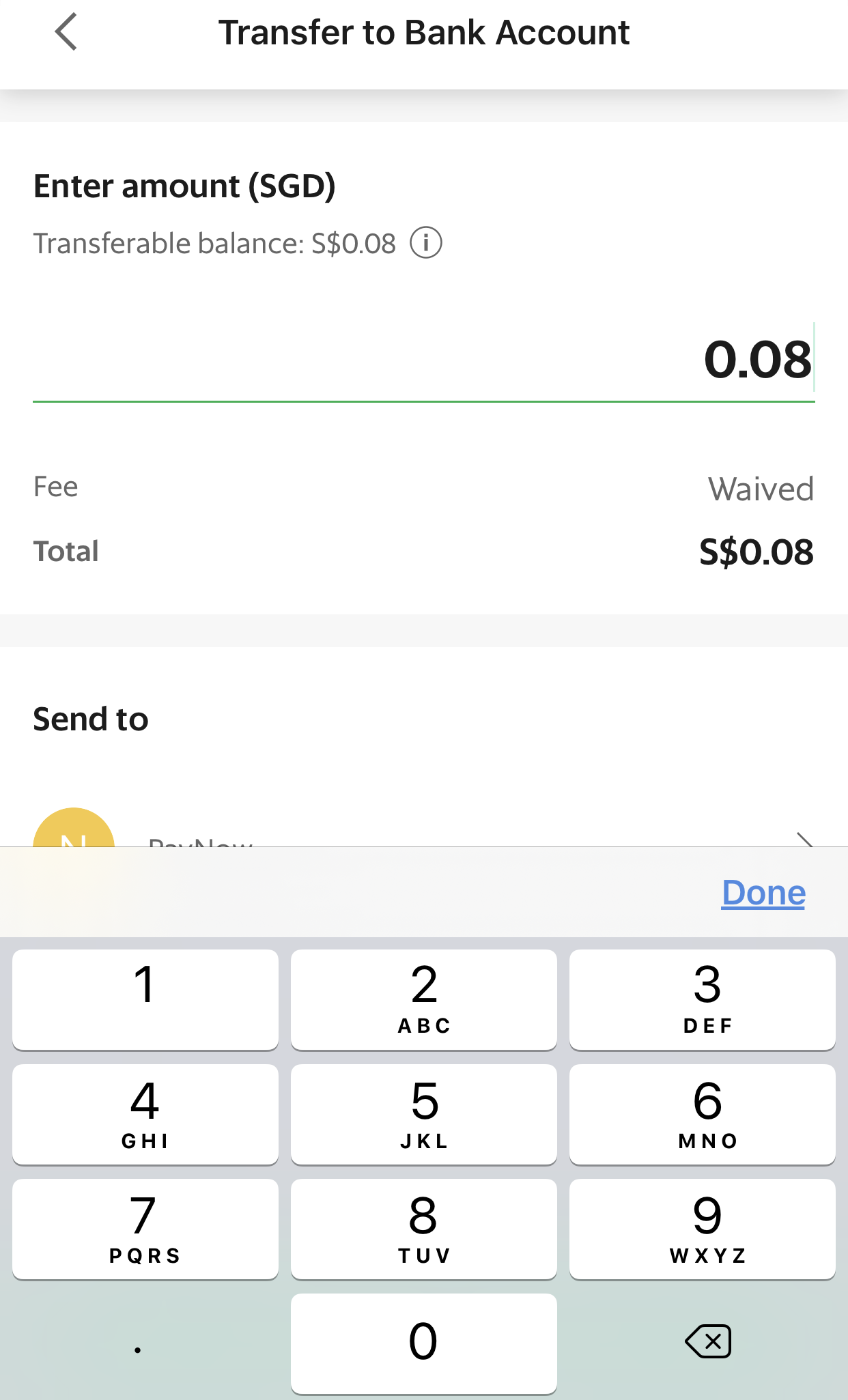The image displays a screenshot from a cell phone or tablet interface showing a bank account control panel. At the top of the screen, there is a left-pointing arrow. Below this, on a white background, is a heading that reads "Transfer to Bank Account." Beneath the heading, on a light gray background, there are fields labeled "Enter Amount," "SGD," and "Transferable Balance." The transferable balance is displayed as "0.08" with an information icon next to it. Below this, the text "Fee is waived" and "Total: 0.08" are shown.

A pop-up keyboard is visible on the screen, featuring numbers 0 through 9, a period, and buttons labeled "Done" (located in the upper right corner) and a backspace button marked with an "X" (in the lower right corner). There is also an "N" on a yellow background, partially obscured by the pop-up keyboard.

In summary, the screenshot captures a banking app’s transfer interface, highlighting a small transferable balance with an active numeric keyboard overlay ready for input.